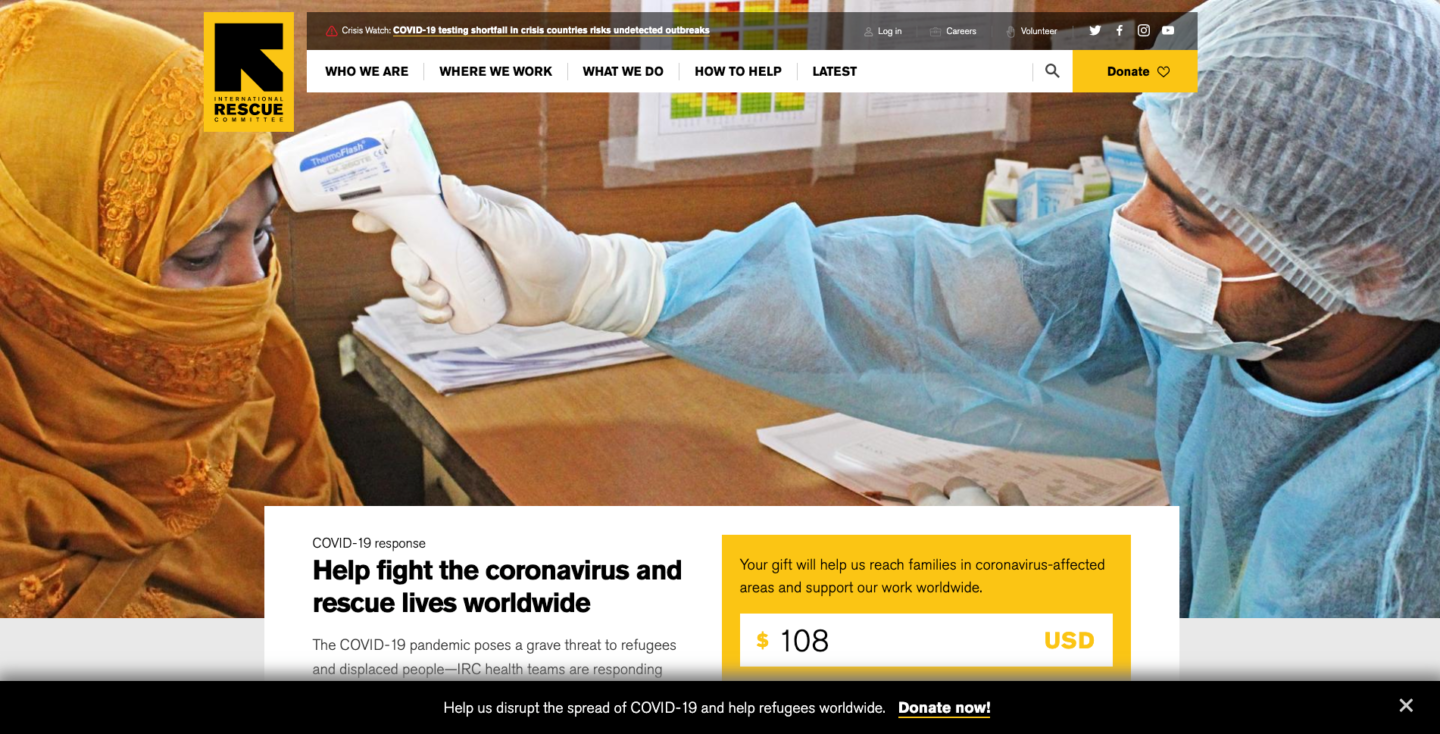A detailed descriptive caption for the screenshot of the website landing page:

---

The image captures a screenshot of a website's landing page dedicated to COVID-19 resources. The large banner prominently displays a compassionate scene depicting a healthcare professional and a patient. On the left side of the banner, a woman wearing a golden-yellow hijab with orange embellishments, which covers her hair and the lower part of her face, reveals only her eyes. She is seated and facing a dark-skinned male healthcare worker on the right side of the banner. The healthcare worker, donning a pale blue translucent hairnet and matching gown, is extending his right arm, which is gloved in white latex, holding a white thermometer gun directed at the woman's forehead, indicating he is checking her temperature.

Above the banner, the website's menu, featuring options like "Who We Are," "Where We Work," "What We Do," "How to Help," and "Latest," provides easy navigation. A magnifying glass icon represents the search function, while a prominent yellow "Donate" button with a black-outlined heart invites visitors to contribute.

Below the banner, a bold black arrow points towards the website title "Rescue" situated in a yellow block. Underneath, a white field with bold black text reads: "COVID-19 resources: Help fight the coronavirus and rescue lives worldwide." This transitions into smaller unbolded black text: "The COVID-19 pandemic poses a grave threat to refugees and displaced people. IRC health teams are responding."

Positioned to the right, a yellow box emphasizes, "Your gift will help us reach families in coronavirus-affected areas and support our work worldwide." Inside the yellow box, a white field displays "108" in black font accompanied by a yellow dollar sign indicating the potential donation amount in USD. Below this, a black bar with white text urges, "Help us disrupt the spread of COVID-19 and help refugees worldwide." A bold white text underlines the urgent call to action with "Donate now" in yellow, underlined.

---

This thorough caption integrates details about the website's design, navigation, visual elements, and the call to action for donations, portraying a clear and vivid understanding of the landing page’s intent and layout.